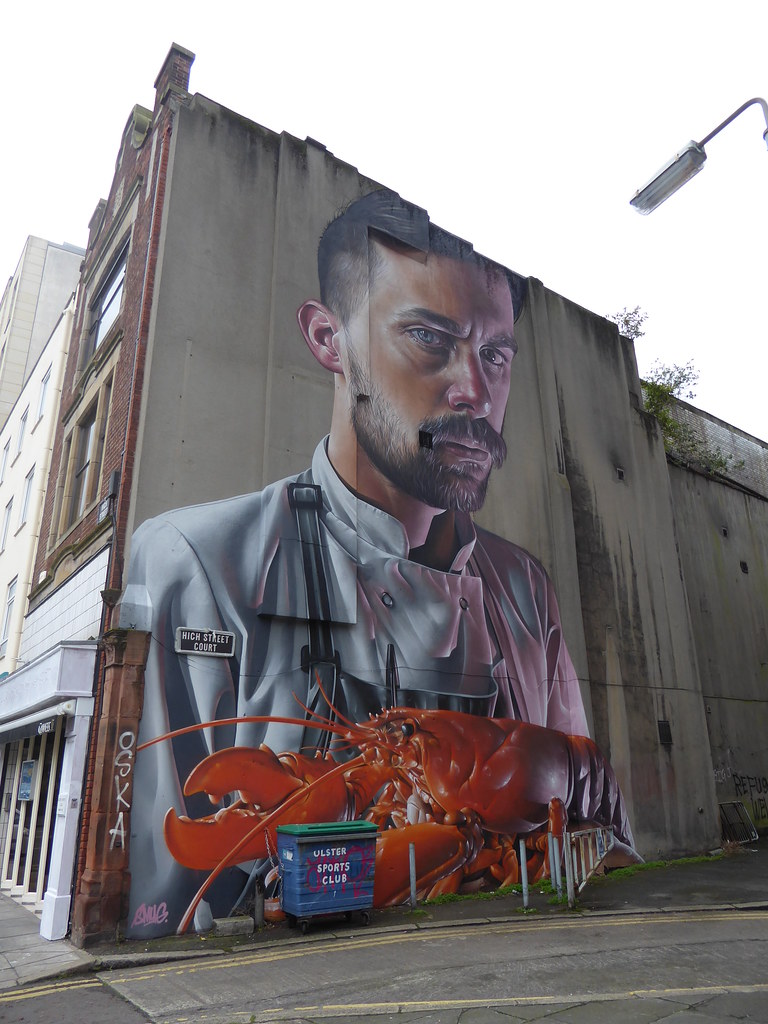This detailed image captures a striking mural on the side of a tall building. The building's main structure is red brick with a gray concrete side where the mural is painted. This photorealistic mural features a man with dark brown hair, a well-groomed beard, a mustache, and a piercing gaze with one blue eye and one brown eye. He wears a white shirt resembling a chef’s uniform, possibly with suspenders and a badge that reads "High Street Court." His expression is serious and focused. Sitting prominently at the bottom of the mural is a large red lobster with distinguishable pincers. In front of the mural, a blue bin marked "Ulster Sports Club" and several parking bollards are visible, with a street running parallel to the building. The streetlight peeks into the image from the top right, adding to the urban atmosphere. The word "OSKA" is noticeable near the mural, contributing an additional layer of graffiti to the artistic scene. The mural is complemented by the minimal view of the storefront and the windows on the building's brick front, creating a vivid and elaborate depiction of this urban artwork.